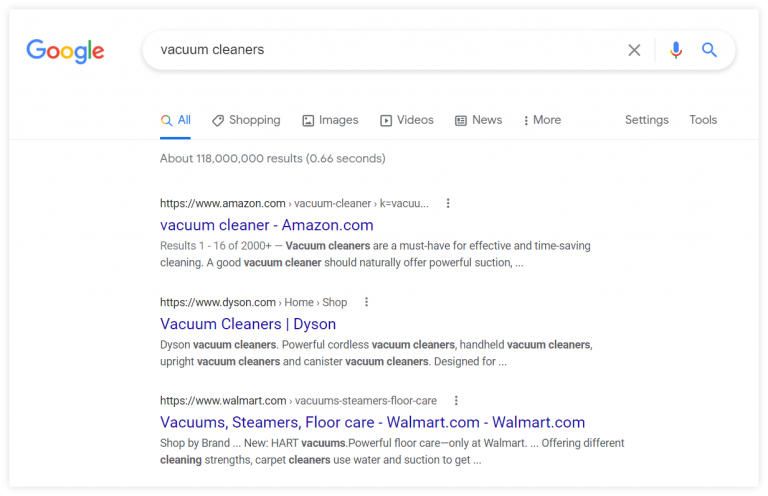A screenshot of Google search results is displayed, focusing on the query "vacuum cleaners." Situated in the upper left corner, the recognizable Google icon is visible. The search bar, under which the query is typed, is set against a white background, with text appearing in black. The "All" tab is selected, highlighted in blue. Additional tabs such as Shopping, Images, Videos, News, and More are also present, alongside Settings and Tools options. The search yields approximately 118 million results acquired in 0.66 seconds.

The first result listed is from www.amazon.com, labeled as "Vacuum cleaner amazon.com," and noted as Result 1 of 220,004. This link emphasizes that vacuum cleaners are essential for effective and time-saving cleaning and suggests that a good vacuum cleaner should naturally provide powerful suction.

The second search result leads to dyson.com, describing various types of Dyson vacuum cleaners, including powerful cordless models, handheld devices, upright vacuum cleaners, and canister vacuum cleaners.

The third result directs to walmart.com, highlighting categories such as vacuum steamers and floor care. It mentions that shoppers can browse by brand and points out Walmart's new powerful Heart vacuum for floor care. This result also briefly discusses carpet cleaners which use water and suction for cleaning.

Although the links are in blue, providing clickable options, the descriptions are generic and lack detailed information about the vacuum cleaners. The suggestion is made that clicking on the Shopping tab might yield more specific product examples, but it’s uncertain if these results are the most informative or beneficial for users seeking detailed information.